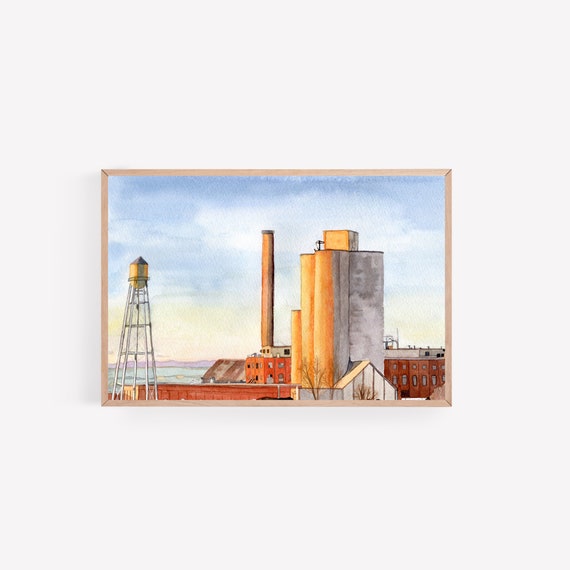The image is a detailed watercolor painting framed in a light brown border, set against a white background. The scene depicts an industrial seascape with a water tower prominently on the left, towering into the midpoint of the painting. The sky above transitions from dark blue to light blue with watercolor clouds, suggesting light from the left.

Centrally, a tall, orange-colored industrial chimney rises higher than the water tower, contributing to the scene's factory-like atmosphere. Adjacent to the chimney is a tall, commercial building, roughly 15 stories high, painted in a palette of orange, yellow, and white hues, though it lacks windows. The lower section of the painting features a washed-out red building, about three stories high, stretching horizontally with a distinct roofline. This red building has multiple levels and windows with a reddish-brown chimney extending from it. The setting is completed with a shoreline and a hint of the ocean in the backdrop, tying together the industrial elements with the seascape.